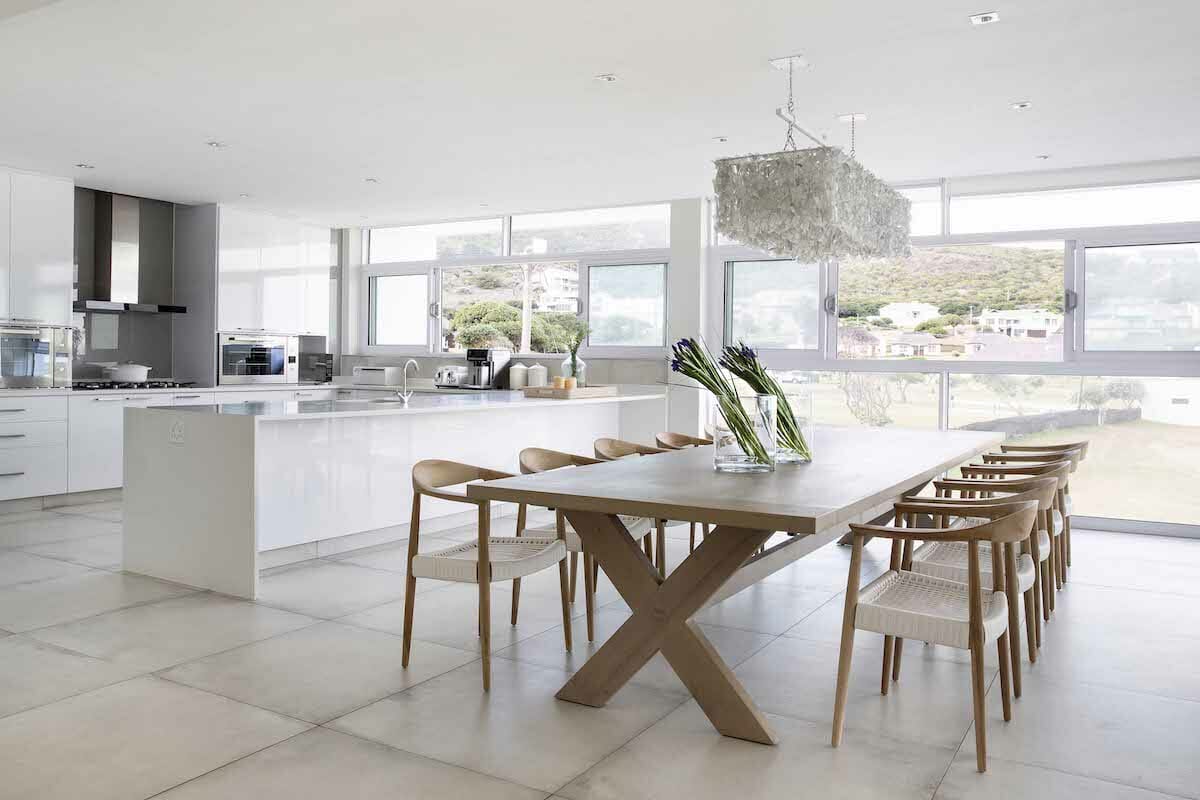The photograph captures a high-end, modern kitchen and dining area within a bright and airy home. The expansive space is predominantly stark white, accentuated by sleek marble tile flooring. A central feature is the long, white dining table supported by X-shaped light wood legs, surrounded by eight minimalist chairs with wooden frames and white wicker seats. Atop the table, two clear vases hold green plants, adding a touch of nature to the pristine environment.

The kitchen boasts a seamless open design, anchored by a substantial marble island equipped with a stainless steel sink and cutting-edge fixtures. Adjacent to the island, a sleek kitchen counter houses a state-of-the-art stovetop beneath a gleaming metal hood range and an over-range. Modern appliances, including a coffee maker, underscore the room's functionality. 

Flooded with natural light, the back wall is a striking feature composed entirely of large windows, enhancing the spacious feel and providing an impressive view. A flat, somewhat low ceiling fitted with recessed lighting adds to the modern aesthetic. Above the dining table, a contemporary chandelier resembling an oblong box with crystal adornments or an art piece fashioned from delicate materials like feathers or cotton, casts a sophisticated glow across the room. This well-appointed space, possibly intended for a real estate listing or an upscale Airbnb, epitomizes luxury and meticulous design.